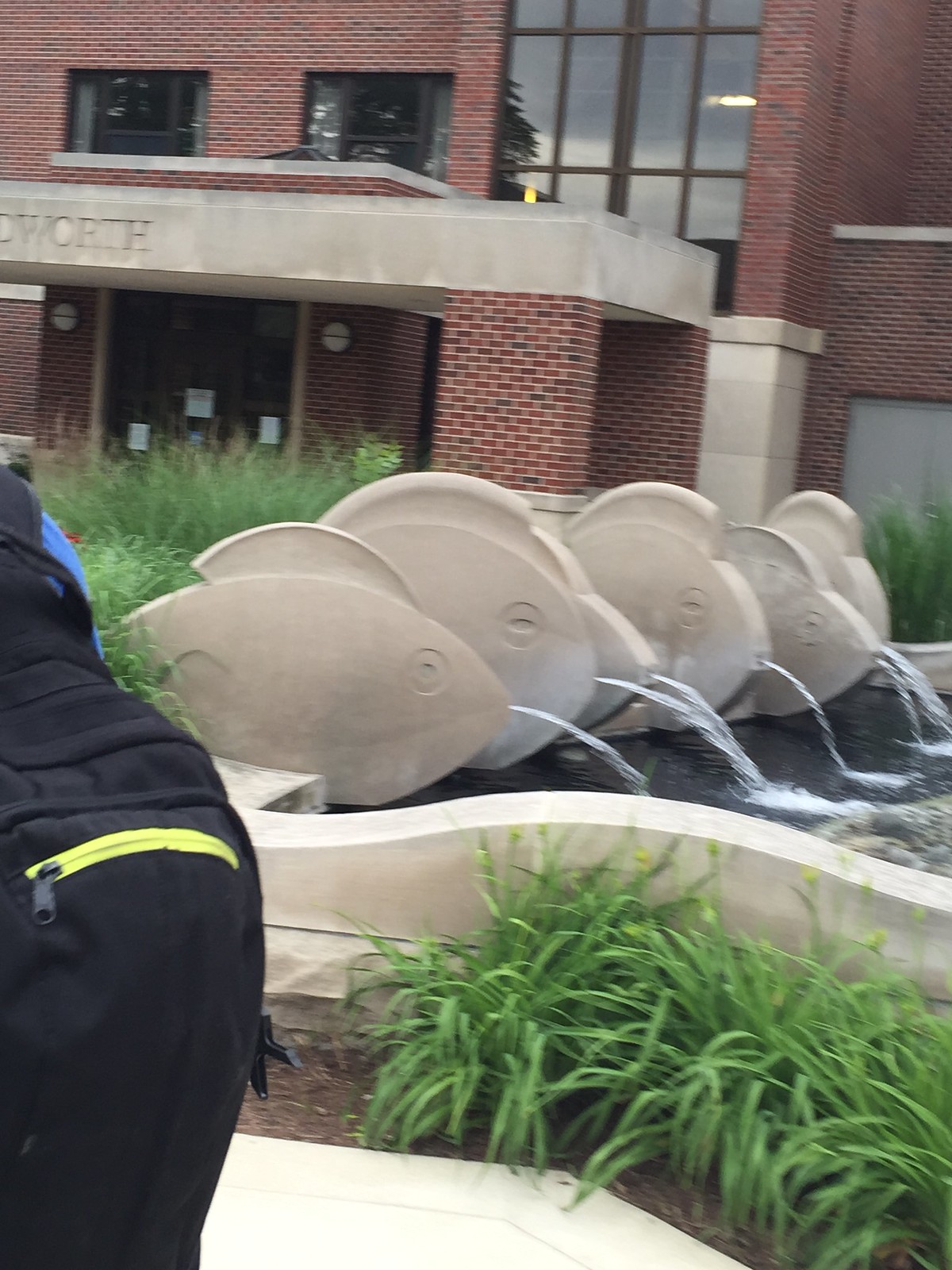In the foreground of the image, an array of five white fish sculptures of varying sizes line an oval-shaped fountain, each spewing water from their mouths. These striking fish are set against a backdrop of lush greenery and carefully landscaped plants that frame the fountain area. A person dressed in black with a blue shirt, possibly a security guard, is visible nearby, underscoring the sense of structure and supervision in the setting. Behind this vibrant scene, a red and brown brick building rises. This building features a flat stone pediment with an inscription partially reading "W-O-R-T-H," supported by brick pillars and adorned with a large cross-hatched glass window, suggesting a multi-storey facility. The tall grasses planted in front of the building complement the shorter grasses lining the fountain, creating a cohesive landscape. A backpack is partially visible in the lower left corner, subtly hinting at human presence and activity in this tranquil space.